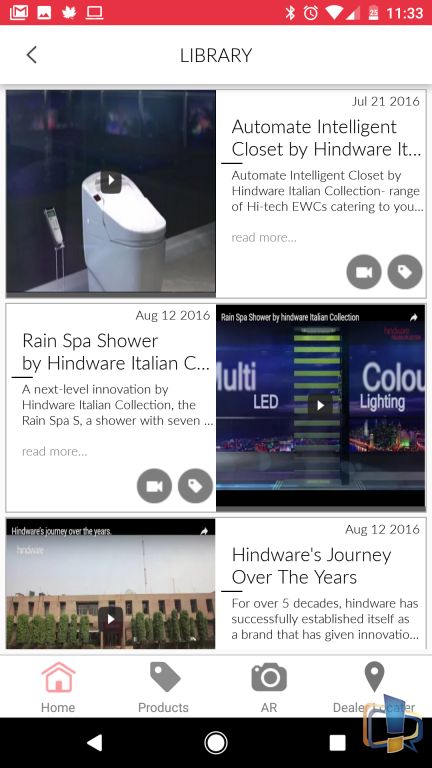**Caption:**

The image showcases a cell phone screen with a detailed user interface. At the top, a red strip contains a Gmail notification on the left, indicated by an email icon, as well as icons for Bluetooth, alarm, data or Wi-Fi, signal bars, and battery level at 25%, with the time displaying 11:33. The main section of the screen has a white background featuring a left arrow on the left side and the word "Library" in the center. Below this, there are two fully visible rows of content boxes, with a third row partially visible.

In the first box on the left, there’s an image of a white appliance that resembles a countertop appliance. The accompanying text reads: "Automate Intelligent Closet by Hindware IT - Automated Intelligent Closets by Hindware Italian collection, a range of high-tech EWC catering to you."

The second box on the left features an image with the text: "Rain Spa Shower by Hindware Italian - A next-level innovation by Hindware Italian collection, the Rain Spa shower with seven…"

On the right side of the screen, both boxes seem to contain videos. The top video shows multi-colored LED lighting that appears to be a sign on the side of a street, set against a possibly black sidewalk. The specifics of these videos are not entirely clear.